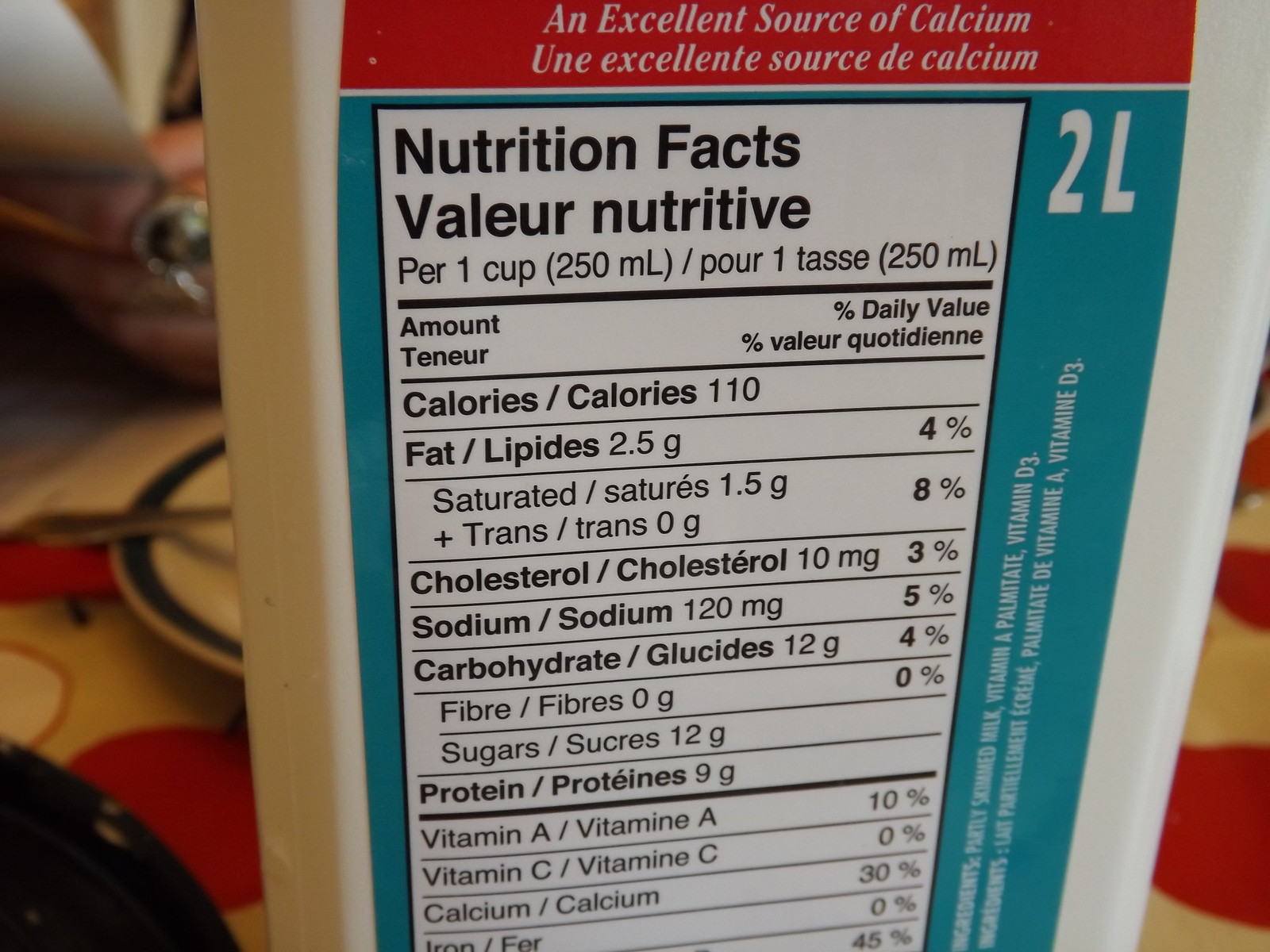The photograph captures the back of a food product bottle. Dominating the frame are the Nutrition Facts, displayed within a white box bordered by black lines. At the top, the header reads "Nutrition Facts" in English and "Valeur Nutritive" in French, indicating bilingual labeling. Detailed nutritional information is listed below, including data on calories, fat, cholesterol, sodium, carbohydrates, protein, vitamin A, vitamin C, and calcium. The bottle itself is white, while the label features a teal turquoise background. A prominent red stripe above the Nutrition Facts highlights that the product is "An Excellent Source of Calcium."